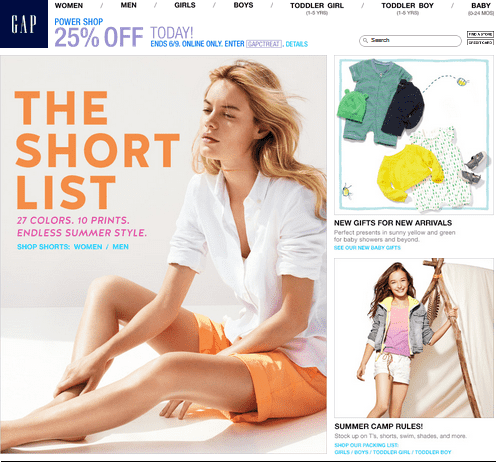The image is a detailed screenshot of the GAPS website storefront. At the top, the website includes navigational sections dedicated to various merchandise categories: Women, Men, Girls, Boys, Toddler Girl, Toddler Boy, and Baby. On the far left corner, the GAPS logo is prominently displayed against a blue background with thin stylized letters spelling out "GAP."

Below the navigation bar, there is a promotional banner mentioning "PowerShop: 25% off today," with additional details such as "N69," indicating the offer is online-only, and a coupon code "GAPSEATREAT" for availing the discount. Adjacent to this is a search bar for users to look up specific items. Some smaller, blurry buttons are situated nearby but are too obscure to identify.

The main content area of the screen is divided into three distinct advertisement sections. On the left, a large ad showcases "Shortlist: 27 colors, 10 prints, endless summer style," inviting customers to shop for shorts available for both women and men. On the right, there are two smaller ads stacked vertically: the top one promotes "New Gifts for New Arrivals," highlighting a range of baby clothes, while the bottom one features "Summer Camp Rules," which showcases merchandise designed for young children preparing for summer activities.